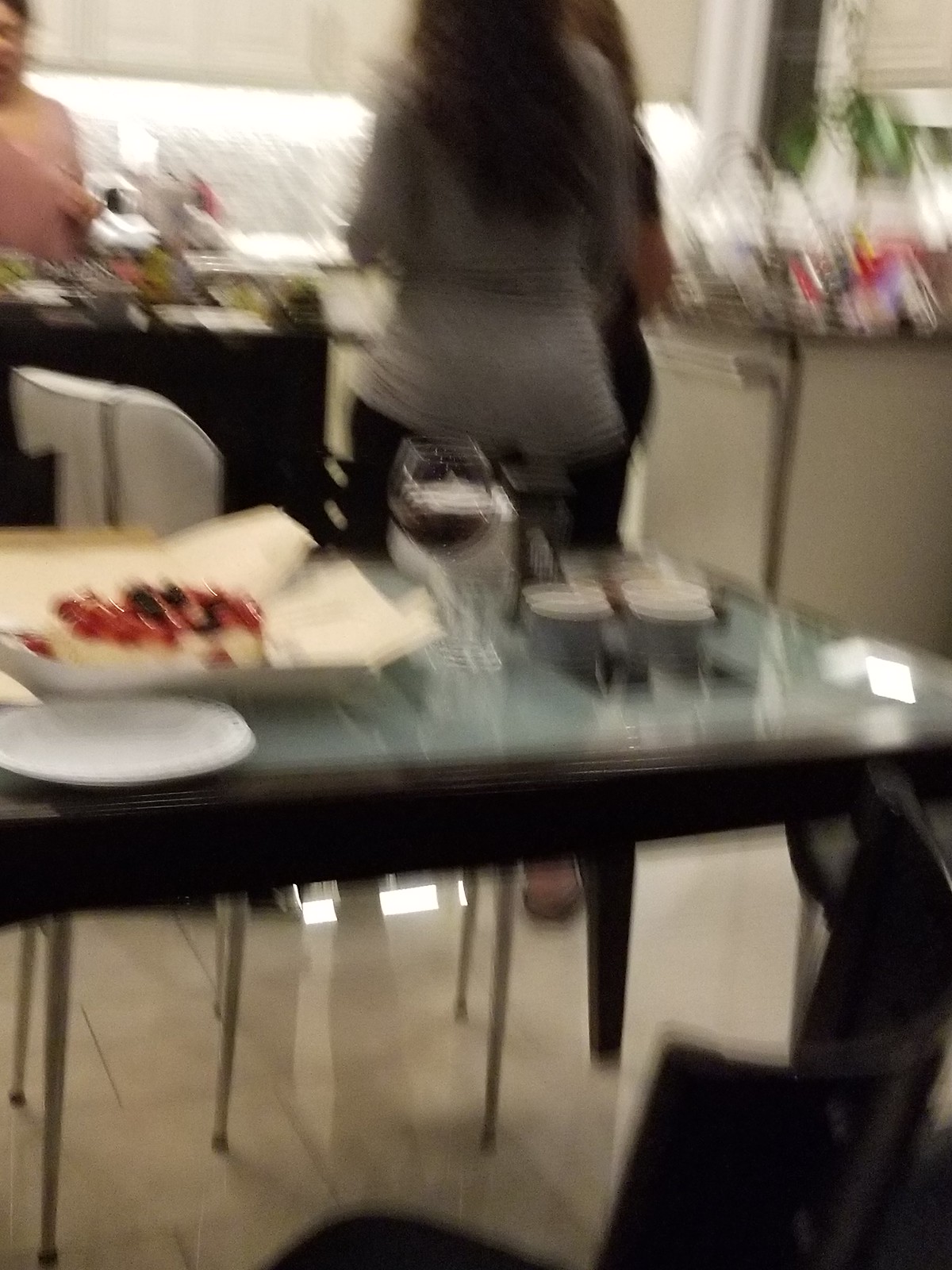This portrait-oriented photograph captures the interior of a cozy kitchen. In the background, white cabinets and a grey backsplash create a clean, modern aesthetic. A kitchen window provides natural light, complemented by a houseplant positioned on the right-hand side, adding a touch of greenery. The foreground features an elegant glass-top table with dark legs and siding, adorned with a variety of items: a fruit-topped cake, a glass of red wine, several plates, and a few cups, suggesting a moment of shared indulgence or celebration. The high-backed chair, matching the table legs in color, is also visible at the very front of the image.

Amidst this domestic scene are three figures. The central figure, located in the middle background, has long, dark hair, and is dressed in a grey long-sleeved shirt paired with black pants. To the left, behind a black counter, stands another person wearing a pink top. There is also a third figure slightly behind the central one, adding depth to the scene.

The image, however, is extremely blurry, as if taken with an unsteady hand, making it difficult to see details clearly. Despite this, the warmth and everyday charm of the kitchen setting are palpable.